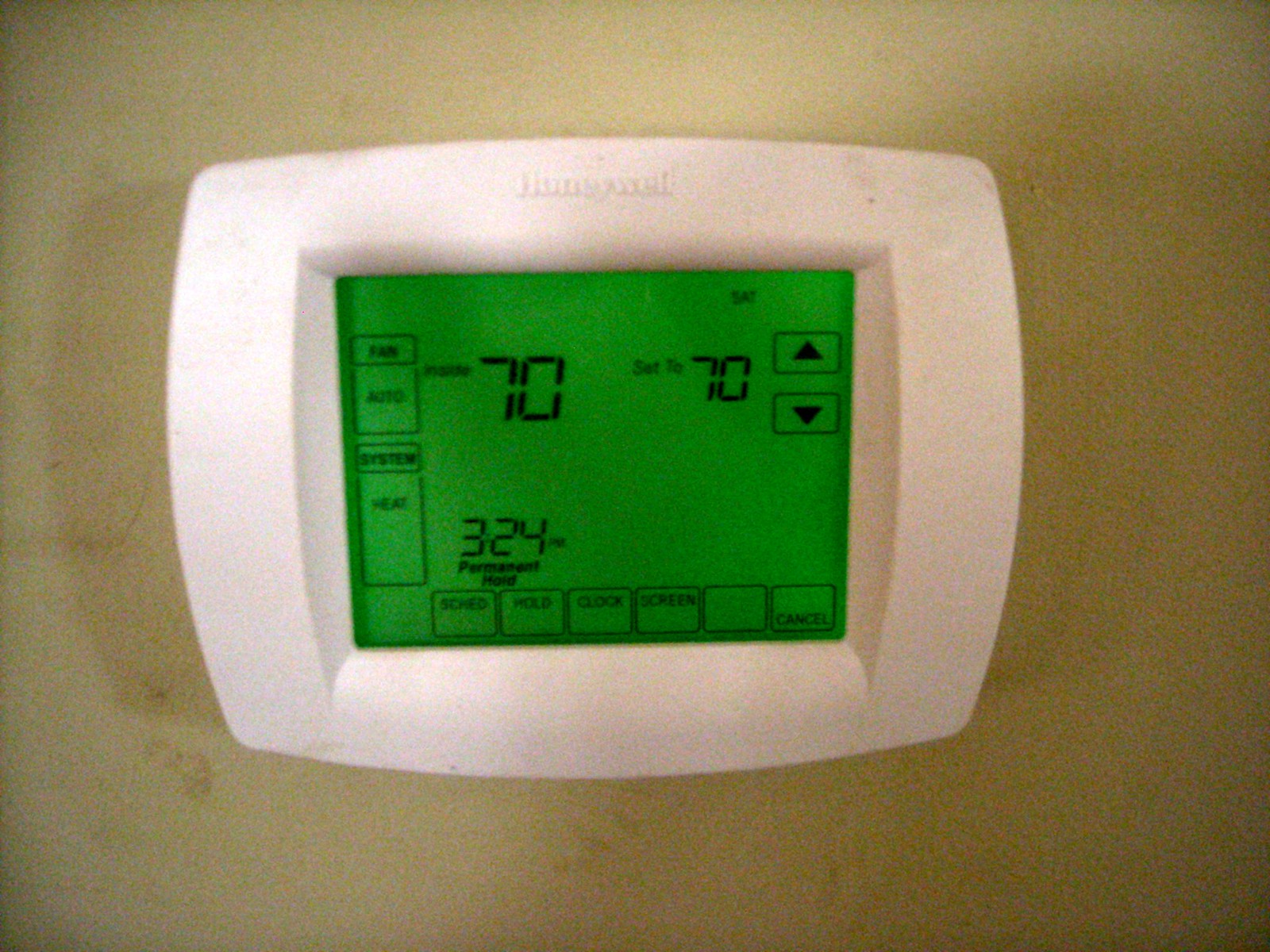This photograph captures a grainy and low-quality image of a wall-mounted thermostat, set against an off-white wall that appears dirty, possibly due to camera artifacts or actual marks. The primary focus is the white, rectangular Honeywell thermostat featuring a fully digital screen devoid of any physical buttons. The screen displays a temperature of 70 degrees next to the word "Inside" and the thermostat is set to 70 degrees. On the right-hand side of the screen, upward and downward arrows are visible, alongside the labels "Fan" and "Auto." The system is currently set to "Heat" mode. At the bottom of the screen, the display reads "3-4 Permanent Hold." Below the screen, a series of buttons are outlined in black against a bright neon green background. These buttons are labeled "Schedule," "Hold," "Clock," "Screen," and a blank button, with the final button in the bottom right corner labeled "Cancel."